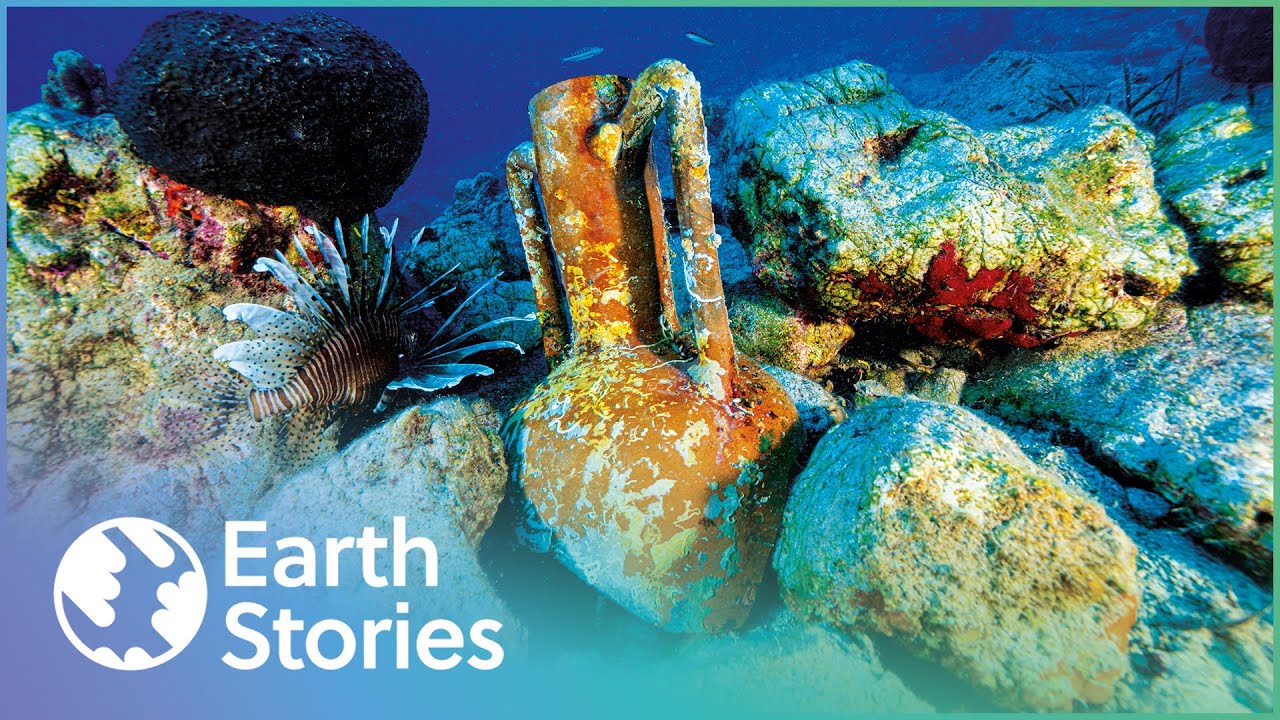Underwater Scene with Rocks, Lionfish, and Ocean Debris

This underwater poster, tinted in teal, depicts a vibrant ocean floor. The scene is anchored by an array of large, weathered white and tan rocks scattered throughout. To the left, there's a distinctive white rock, crowned by an oblong black stone. Adjacent to it, a striking lionfish, adorned with black-and-white stripes and light blue fins, swims gracefully. Below this, another white rock adds depth to the scene.

Centrally placed is the peculiar centerpiece: a rusted, orange-and-white metal object. Resembling an upside-down hammer or mallet with a thick cylindrical top and handle-like protrusions, it stands out amongst the natural elements. More large rocks continue to the right, leading up to a series of flat, white stones ascending from the bottom corner to the top, blending into the distant blue water which harbors more fish and submerged rocks.

In the bottom left corner of the poster, there is a simplified white round logo with a blue symbol inside, next to the bold white text "Earth Stories," anchoring the viewer's attention to the thematic essence of the image.